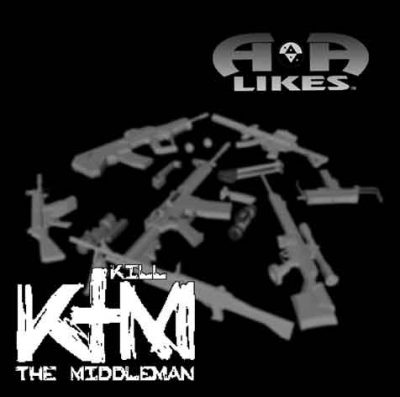The image appears to be a poster or cover related to a game, with a solid black background. At the top right corner, a logo comprising two back-to-back A's is present, with the word “LIKES” beneath it and an icon featuring upside-down and right-side-up periods in black and white. Central to the image, there is an array of gray rifles, machine guns, AK-47s, Sten guns, snipers, and semi-automatic firearms, arranged in a random, flat, almost toy-like manner, devoid of highlights or lowlights. The lower left corner features the heading "KILL K + M" in white, stylish designer fonts, with the ‘T’ resembling an upside-down cross. Below this, there is text stating "The Middleman," further enhancing the stylized and thematic presentation of the poster.